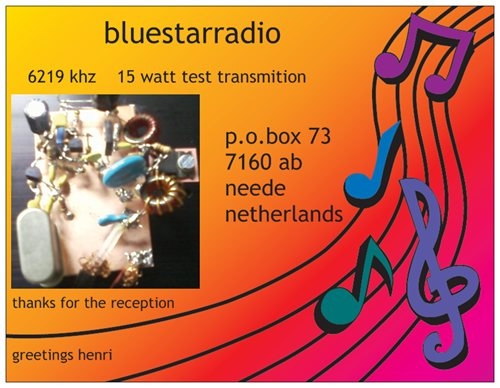This image is of a postcard or flyer for Blue Star Radio. The postcard features a gradient background that transitions from mustard yellow in the top left corner to a magenta pink in the bottom right. Printed in bold black text at the top of the card is "Blue Star Radio," followed by "6219 kilohertz, 15-watt test transmission." Below this text is a photo displaying the interior components of an electronic device, including wires, capacitors, and other small parts. Beside this photo, centered on the flyer, is the address: "P.O. Box 73, 7160AB, Neede, Netherlands." A message below the photo reads "Thanks for the reception," with a closing note saying, "Greetings, Henry," located in the bottom left corner. Along the right edge of the postcard, running from the top to the bottom, are several animated music notes in purple, blue, green, and teal, along with a blue treble clef. Black wavy lines traverse diagonally from the bottom left to the top right, adding a dynamic touch to the overall design.